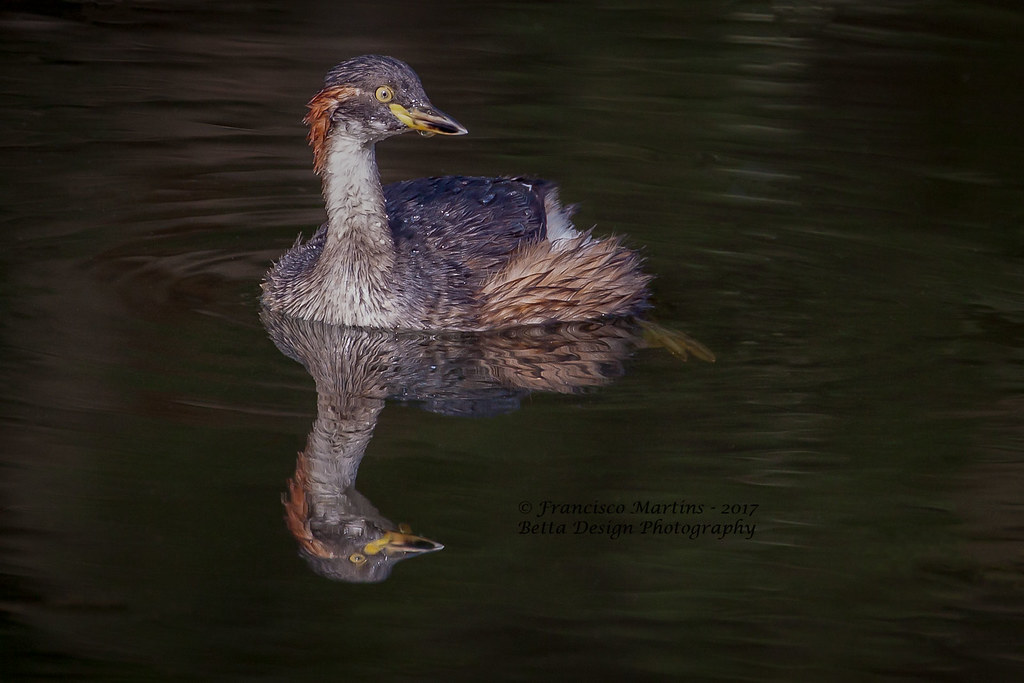This detailed photograph captures a duck floating on dark water, with the entire scene reflected below it. The duck, depicted prominently and slightly off-center, showcases a striking mix of colors: a yellow and black beak, vivid yellow eyes, and a head with a gray hue. Its neck transitions from gray to white, while the back and body exhibit a blend of brown, black, and light gray feathers, gleaming wet from the water. A distinctive red streak adorns the back of its neck, adding a touch of vibrant contrast. The water, calm with subtle ripples, bears the duck’s mirror image and is overlaid with black text indicating the photograph's professional nature. This text reads, "Francisco Martins, 2017, Beta Designs, Photography," confirming the image’s authorship and date.